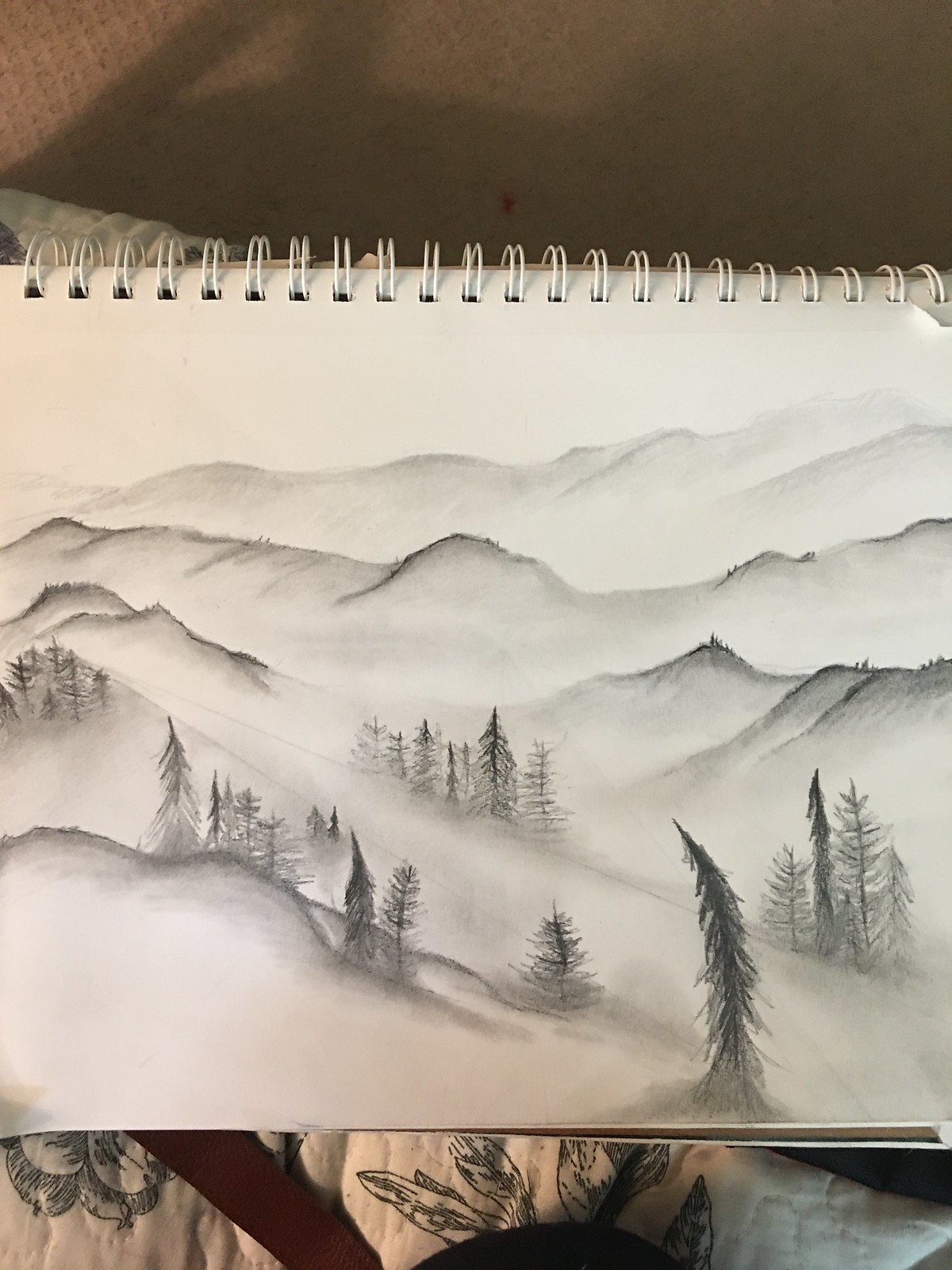This detailed photograph captures a sketchbook placed on a soft, patterned fabric surface. The sketchbook, bound with white spirals, lies open to reveal a meticulously drawn landscape executed in black pencil on white paper. Other pages of the sketchbook are visible, adding a sense of depth to the image. The background consists of soft white fabric adorned with a subtle black design. Ambient lighting casts gentle shadows on the fabric. The penciled artwork showcases a mountainous terrain with well-defined peaks, some of which are accentuated with darker shading. Scattered groups of lush and detailed trees add texture to the scene. In the foreground, a tree with a distinctively bent appearance stands out, adding character and depth to the composition.